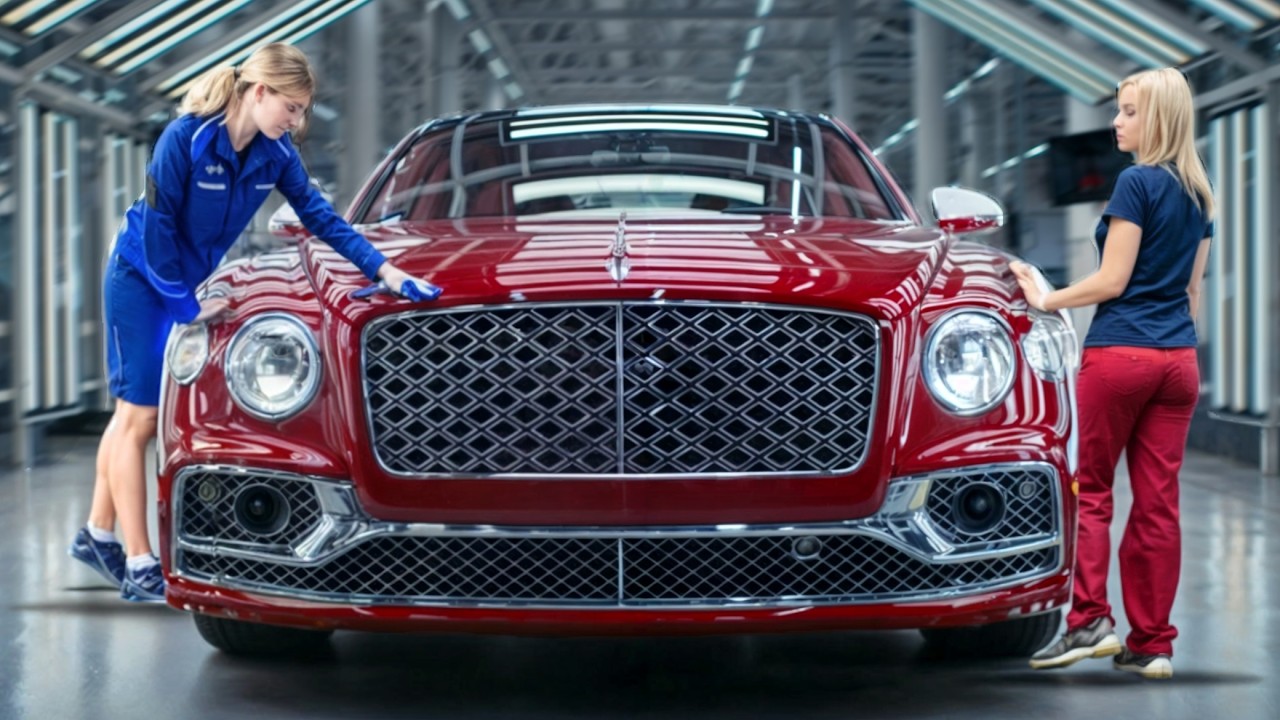The photograph captures a brightly lit factory or showroom interior featuring a blue Bentley luxury vehicle stationed front and center. Positioned towards the bottom left, the car faces downwards with its back door ajar. A blonde woman in a white face mask stands behind the open door, her black shoes visible. On the opposite side of the car, a man with dark black hair and a black face mask leans in, dressed in a black shirt adorned with a white patch across the chest. In the bottom right corner, a woman with red hair cascading down to her shoulder, wearing sunglasses, looks to the left. She sports a very tight green tank top featuring the Bentley logo in black letters over her right breast and khaki pants, with her hands resting near her hips and a hint of her stomach showing. Behind the blue Bentley, a white car is directly visible, followed by several darker-colored vehicles. The ceiling and walls are fitted with sections of three long fluorescent lights, divided by white bars descending from the roof, illuminating the entirety of the facility.